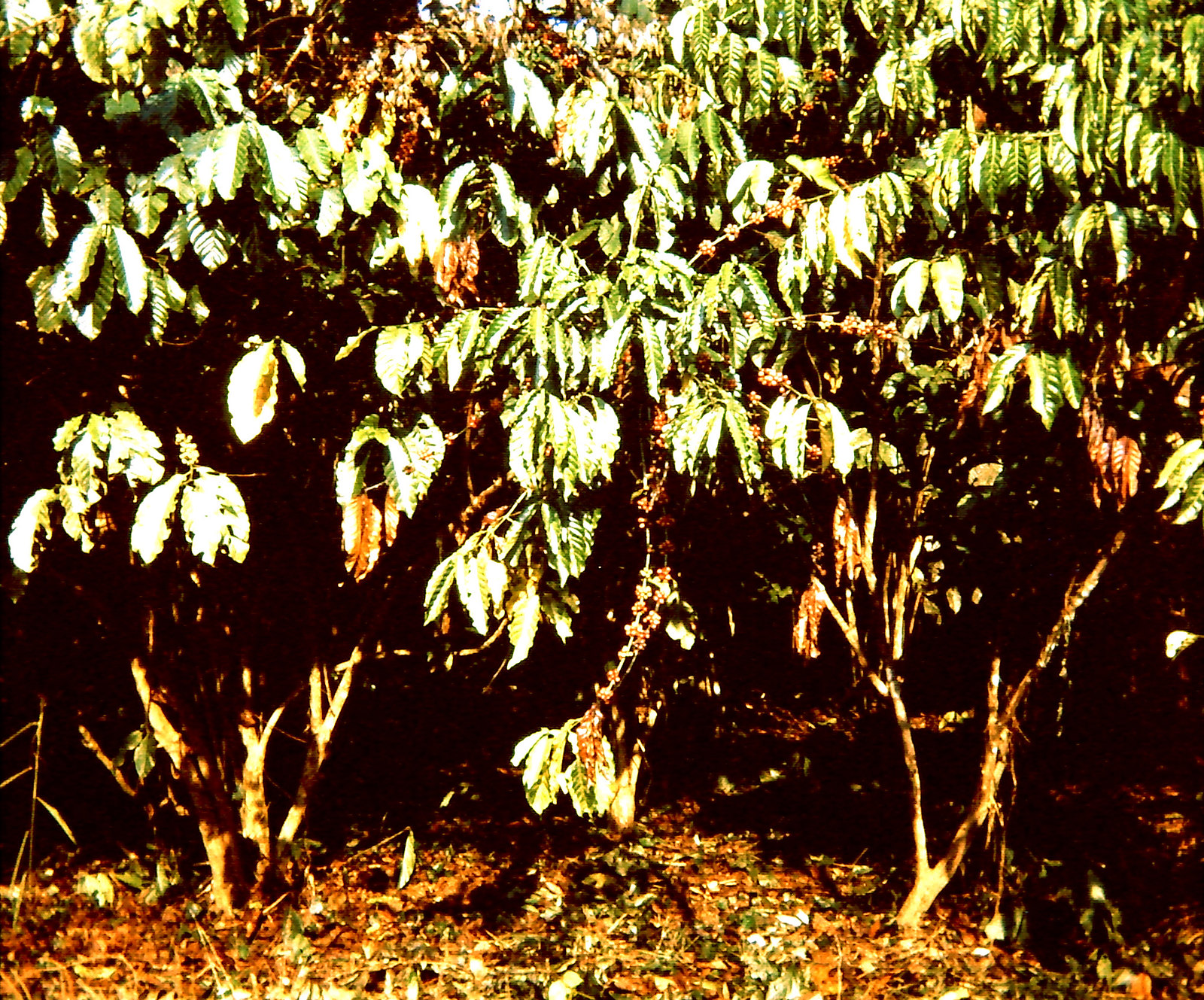In this overexposed, somewhat grainy photographic image, the setting is an outdoor daytime scene featuring a patch of low-lying vegetation. The central focus is a small branch or bush with green leaves, interspersed with about six or seven orange blossoms that run down the center of the foliage. The overexposure renders the colors intensely bright, making the greens appear almost white. The leaves on the bushes have a long, teardrop shape, similar to peach leaves. The branches are low to the ground, creating a dark, shaded area underneath that suggests a canopy-like cover over the forest floor. Scattered around the foreground are numerous leaves in various stages of decay, in shades of brown, orange, and green. The background shows a dull, gray sky blending into a forested area, adding to the overall impression of an old, slightly blurry photograph, possibly evoking a vintage feel from decades past.